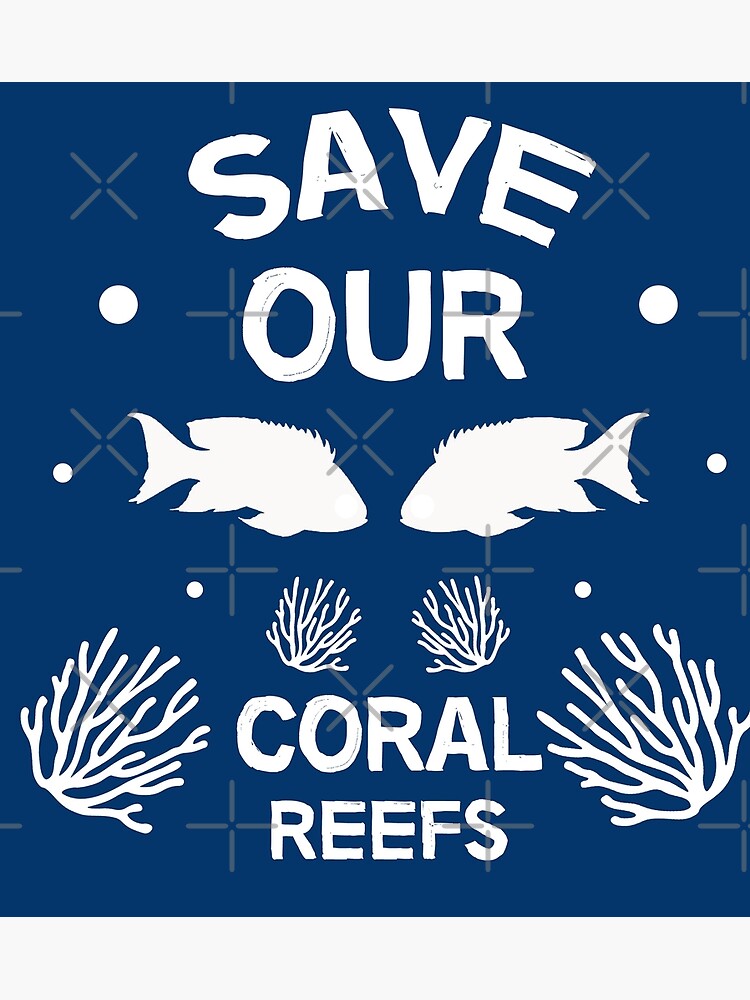This poster, designed to promote awareness about saving coral reefs, features a striking and simplistic layout with a dark blue background. Dominating the top and middle sections of the poster are large, bold white letters spelling out "Save Our Coral Reefs." Interspersed within the text and spread throughout the background are small white circles and silver-gray X and plus sign shapes, which add texture and visual interest to the design. 

Central to the imagery are two white silhouetted fish with spiked scales and large back fins, positioned to face each other as if they are about to kiss. Surrounding the text "Coral Reefs" at the bottom are four pieces of white coral, strategically placed to create balance: two smaller corals just beneath the fish's mouths, and two larger ones flanking the text. The clean, minimalistic design of the poster effectively communicates its environmentalist message, urging viewers to take action in protecting the ocean's vital coral reefs.